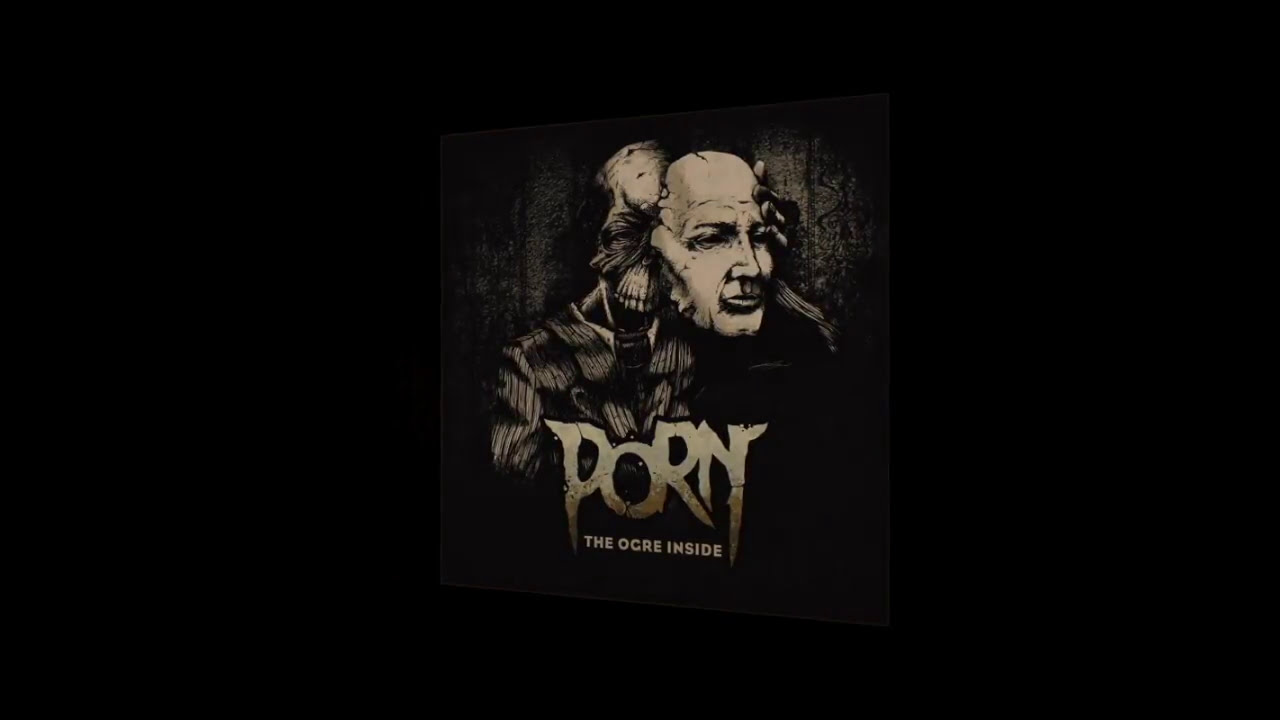The image is a dark, eerie movie poster set against a completely black background, which makes the central sepia-toned and copper-tinged drawing stand out starkly. Dominating the center is an unsettling, older-looking bald man with prominent wrinkles, dressed in a light gray and black pinstripe suit. His face, turned towards the right, reveals a solemn and creepy expression. Perched on his right shoulder is a mysterious, mouse-like or monkey-like creature, adding to the macabre atmosphere. The title "PORN" is prominently displayed in a bold, graffiti-like gradient font, seeming to drip downward. Just below in a smaller, neat font, possibly Arial, is the subtitle "The Ogre Inside."